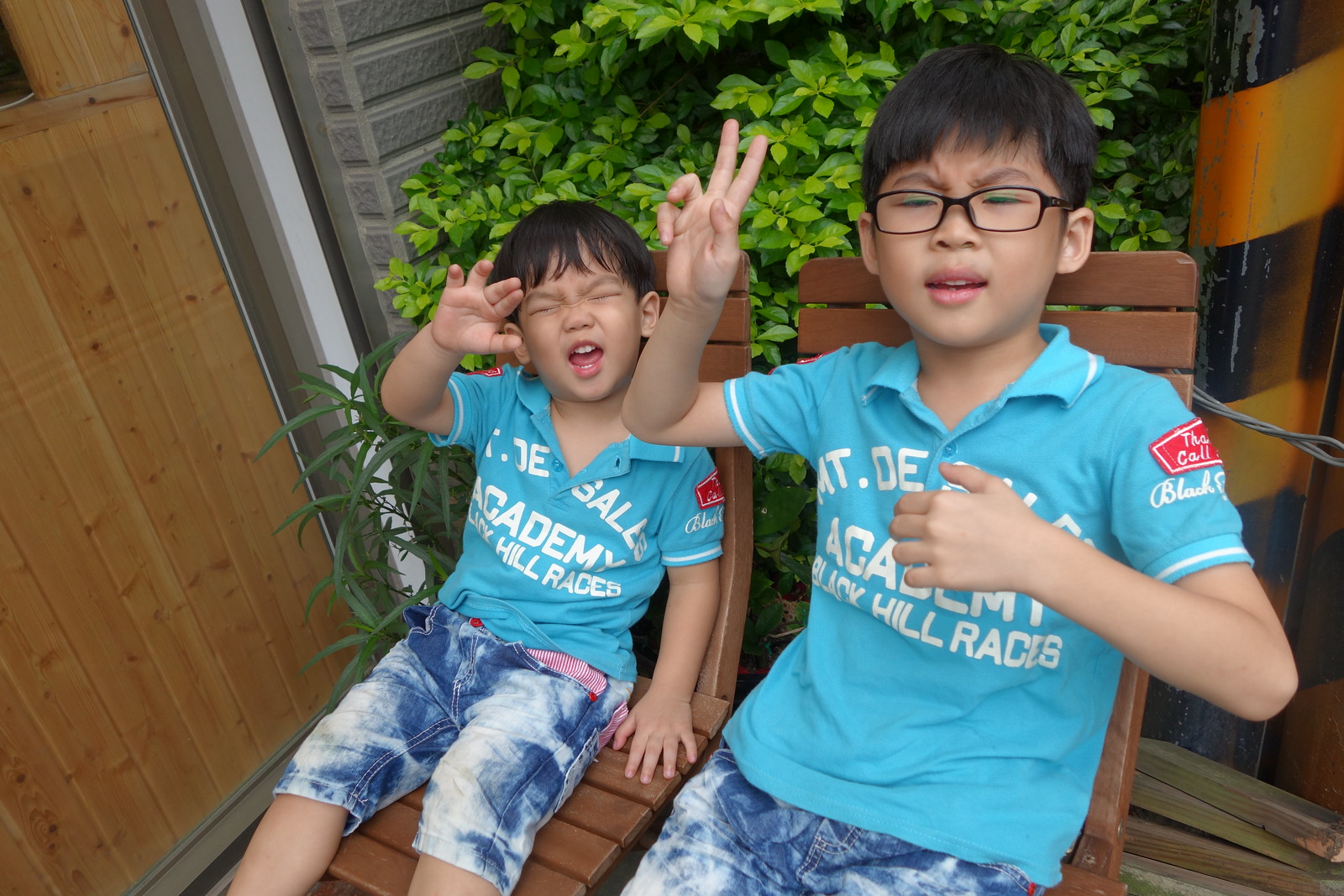Two little boys are sitting on brown wooden chairs in front of a house. They are both dressed in identical blue Academy Hill t-shirts and matching jean shorts that feature a bleached effect, blending blue and white. The boy on the left has his eyes squinted and mouth open, raising all five fingers on his right hand high in the air. The boy on the right wears black glasses and has a more reserved pose, flashing a peace sign with his right hand while his left elbow is bent, hand close to his chest. Behind them, there is a glimpse of a bush and what appears to be a sliding glass door or window. Despite their different gestures, both boys look happy and animated, celebrating something together.